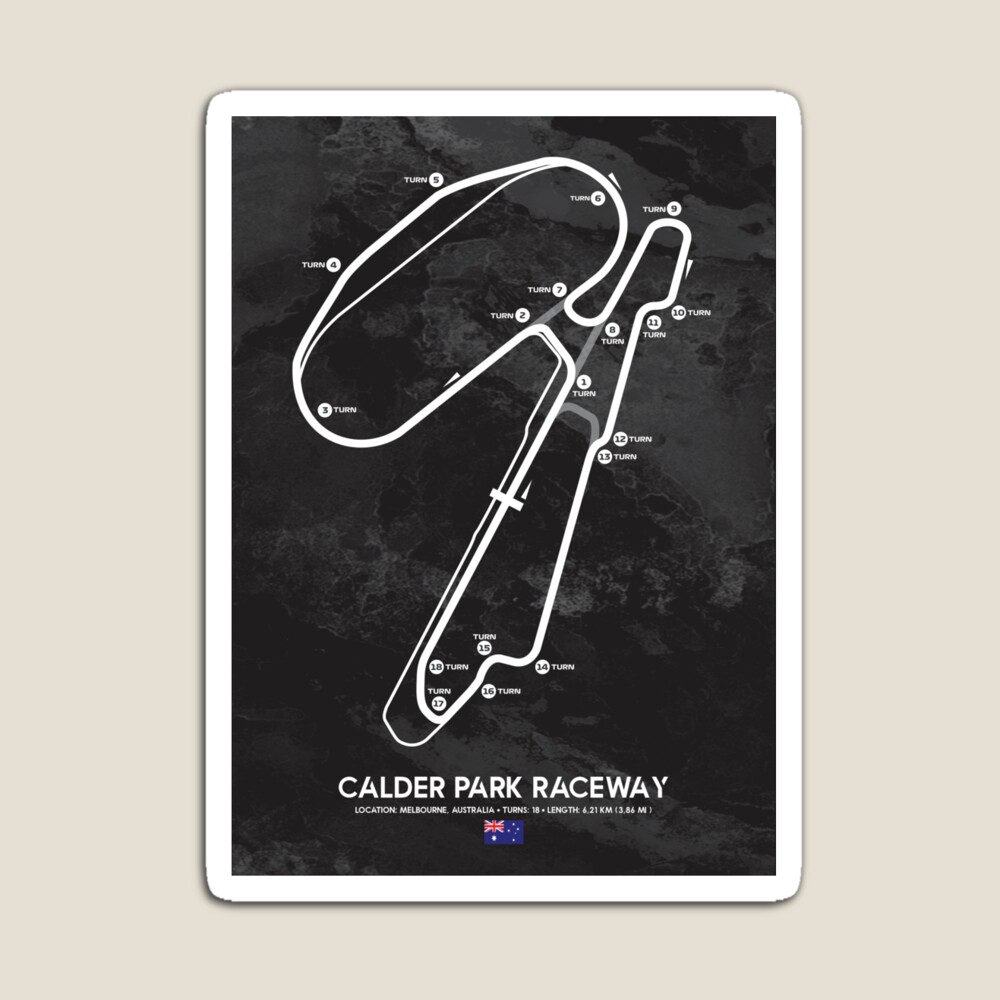The image is a detailed poster of Calder Park Raceway located in Melbourne, Australia. The poster features an illustrated layout of the racetrack in white on a black background, with each of the 18 turns labeled and marked with numbers. The total length of the track is specified as 6.21 kilometers (3.86 miles). Surrounding the poster is a white border, and beneath the track layout, there is text indicating the racetrack’s location and specifications. Additionally, an Australian flag is displayed below this information. The background outside the poster is a light green color, making the detailed and colorful elements of the poster stand out prominently.